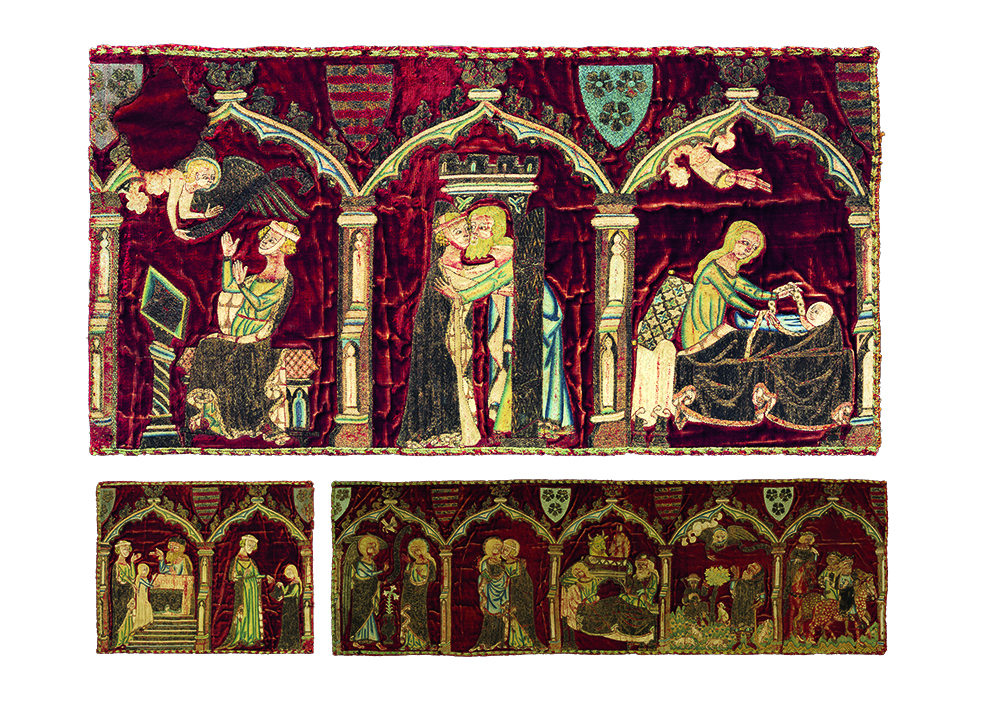The image showcases a richly detailed vintage tapestry with an overall color scheme of red and gold, illuminated brightly by natural lighting. The tapestry is divided into multiple panels, each depicting intricate scenes. The top half of the tapestry dominates the image and features three main scenes: in the center, a man and a woman are depicted hugging; to the right, a woman holds a baby laying down on a bed; on the left, a seated figure extends his hands towards a floating being. The background of all these scenes is a deep red adorned with gold accents.

Below the main panels, the tapestry continues with two additional sections of the red fabric. On the left side of the lower section, a group of five people are engaged in various activities, while the right side features a slightly larger panel, divided into five smaller scenes, illustrating additional narrative moments. The entire tapestry is free from any textual elements or numbers, focusing solely on its vivid imagery and historic charm. The overall clarity of the fabric's intricate details is remarkable, underscored by the tapestry's well-preserved condition despite its antique appearance.